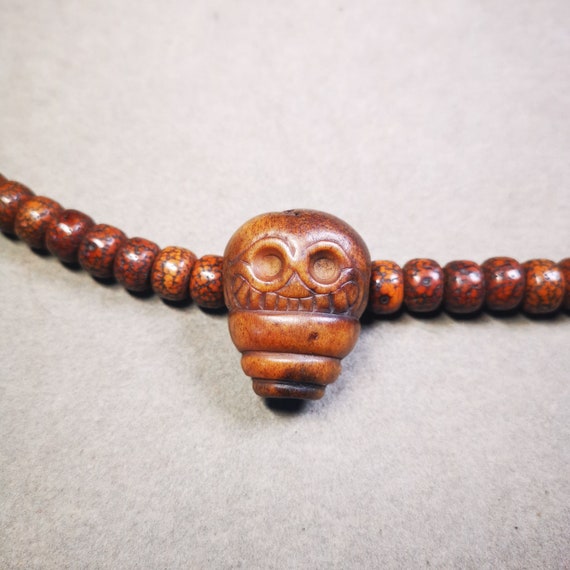This image showcases a detailed, handcrafted wooden necklace, positioned on a textured white surface that has some faded black markings. The necklace is constructed from a series of round and donut-shaped beads in varying hues of brown, orange, yellow, and red, with some beads featuring darker spots or textures. At the focal point of the necklace, there is an intricately carved wooden charm resembling a skull. This charm displays two circular indentations representing eyes, a set of teeth beneath the eyes, and smooth surfaces on the head, giving it a distinctive mask-like appearance. The charm appears to be a dark brown wood, complementing the earthy tones of the surrounding beads.